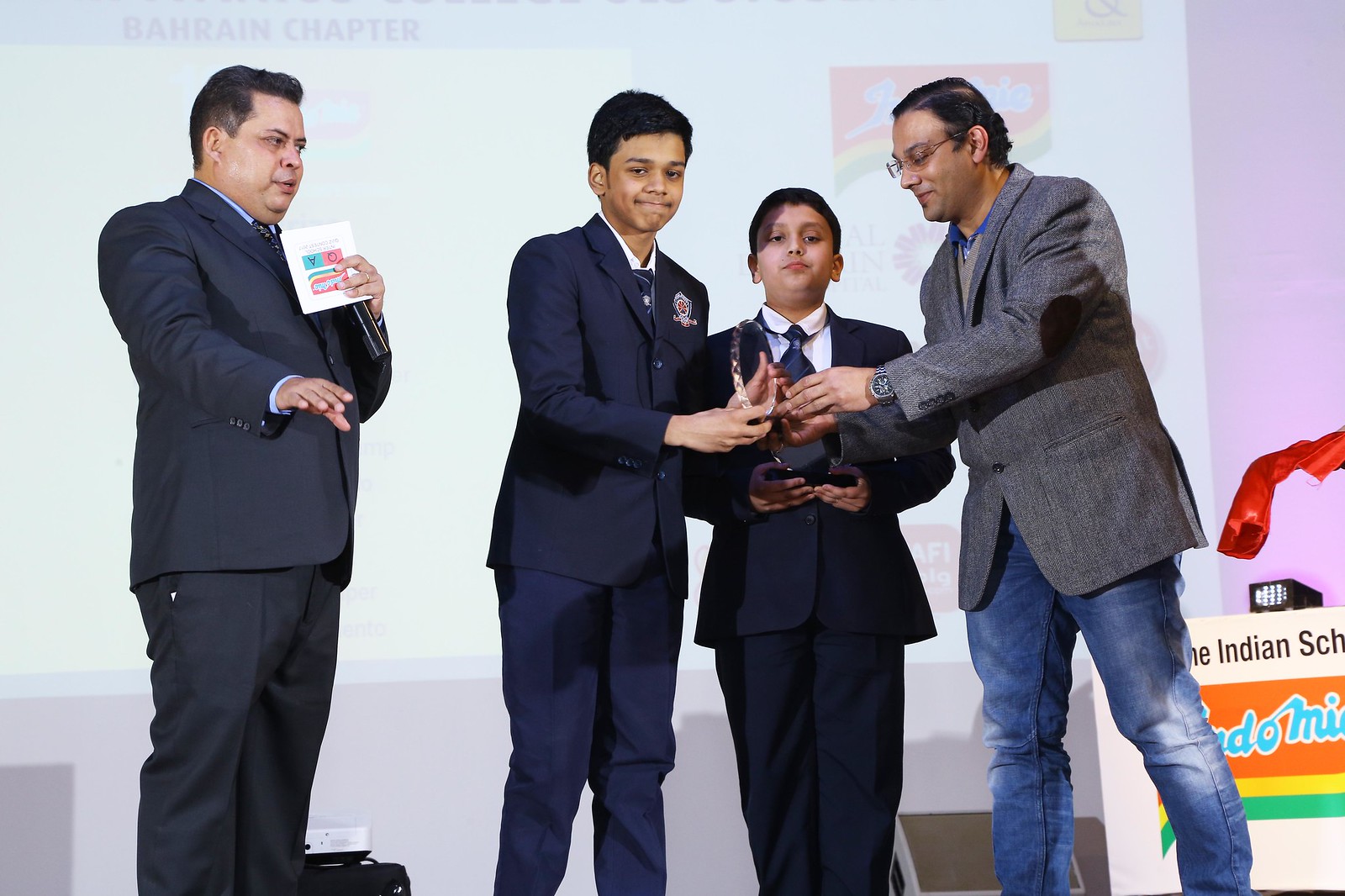On a stage in India, four individuals stand under a faintly projected screen. On the far left is a heavy-set older man in a dark navy blue suit, holding a microphone and gesticulating with his hand, appearing to speak. Next to him are two young boys, or teenagers, wearing school uniforms consisting of blue blazers adorned with emblems. Both young men are smiling and each holds a thin, half-foot high glass trophy on a black base. The boy on the right is accepting his award from an older gentleman, who wears a gray jacket and blue jeans, giving off a professorly vibe. The group seems to be at a ceremony, celebrating an achievement, while the projected backdrop faintly displays the words "Indian school."